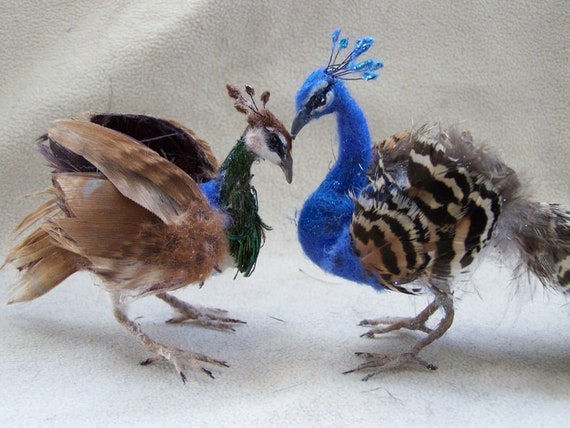This photograph depicts two intricately crafted stuffed peacocks, standing on a white surface against a white background. Both birds are facing each other, creating a striking visual interplay of colors and textures. Despite their realistic appearance, these peacocks are not taxidermy but rather made from materials resembling felt and foam, contributing to their vibrant hues and detailed plumage.

The peacock on the left showcases a harmonious blend of brown and green. The bird's neck features lush green feathers, transitioning to a blue spot on the back and a white patch on its face. Striking black marks encircle its eyes, and it has brown feathers down the center of its head, with additional brown and black stripes cascading over its body. The crest is adorned with brownish feathers, adding an authentic touch.

The peacock on the right contrasts beautifully with a predominantly bright blue head, neck, and chest. Black and white stripes adorn its wings, which are primarily tan feathers. Vivid blue plumes emerge from the top of its head, enhancing its elegant composition. Both birds' legs and talons are visible, further grounding their realistic portrayal. The material and craftsmanship result in a lifelike yet artistic representation, making these peacocks a captivating piece of decorative art.